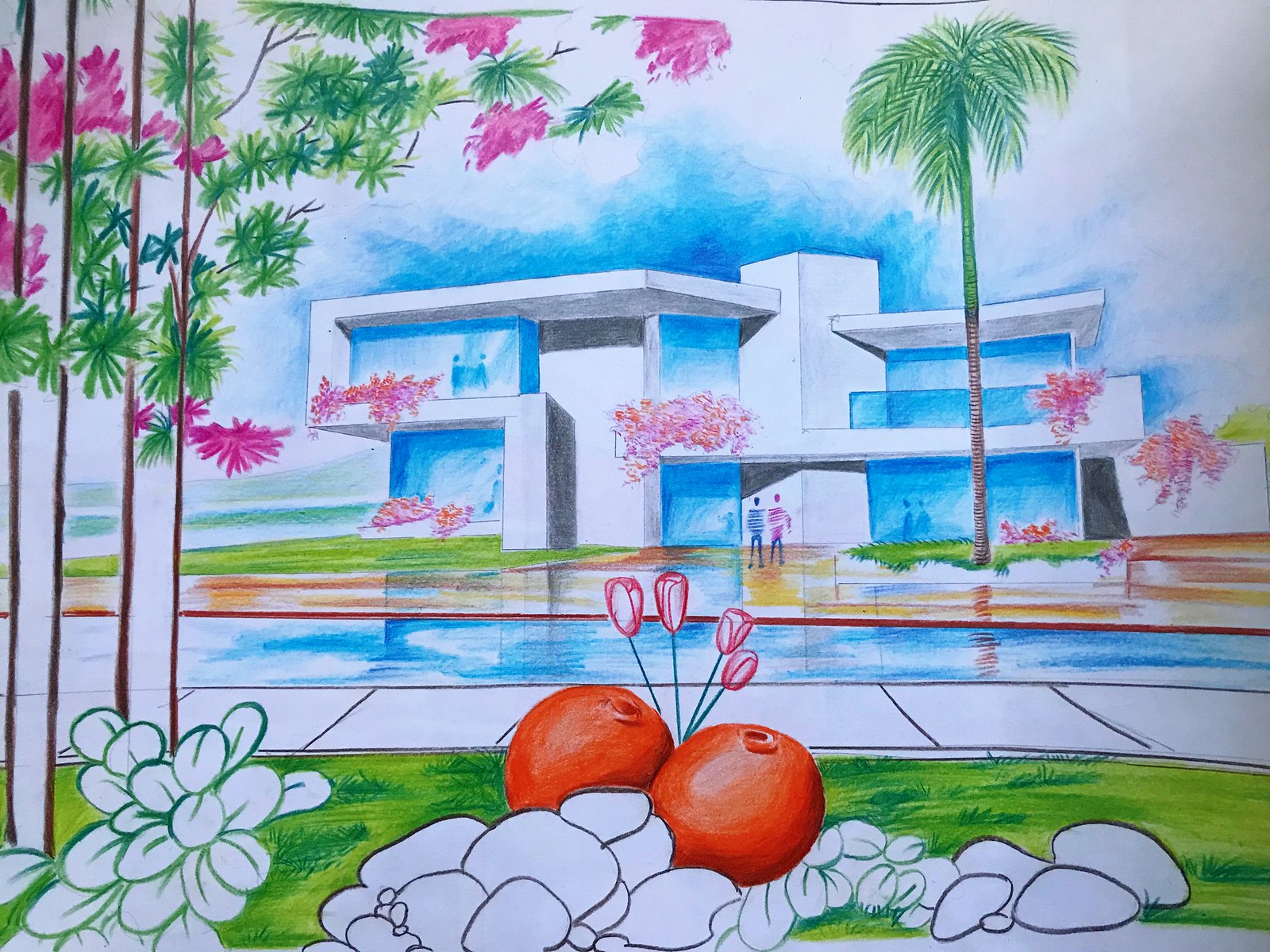This watercolor painting appears to be a conceptual design for a modern building. The scene features a vivid green lawn interspersed with unpainted white rocks and a white bush outlined in green. In the foreground, a pristine white sidewalk borders a tranquil pool that reflects both a towering palm tree and the building itself. To the left, lush trees adorned with green leaves and pink flowers frame the composition. The building at the center is a two-story structure characterized by sleek, modern architecture. Its exterior is a mix of extensive blue glass windows and crisp white walls. Pink flowering bushes drape gracefully from the balconies, adding a touch of natural elegance to the contemporary design. The sky above is mostly cloudy, casting a diffused light over the entire scene.